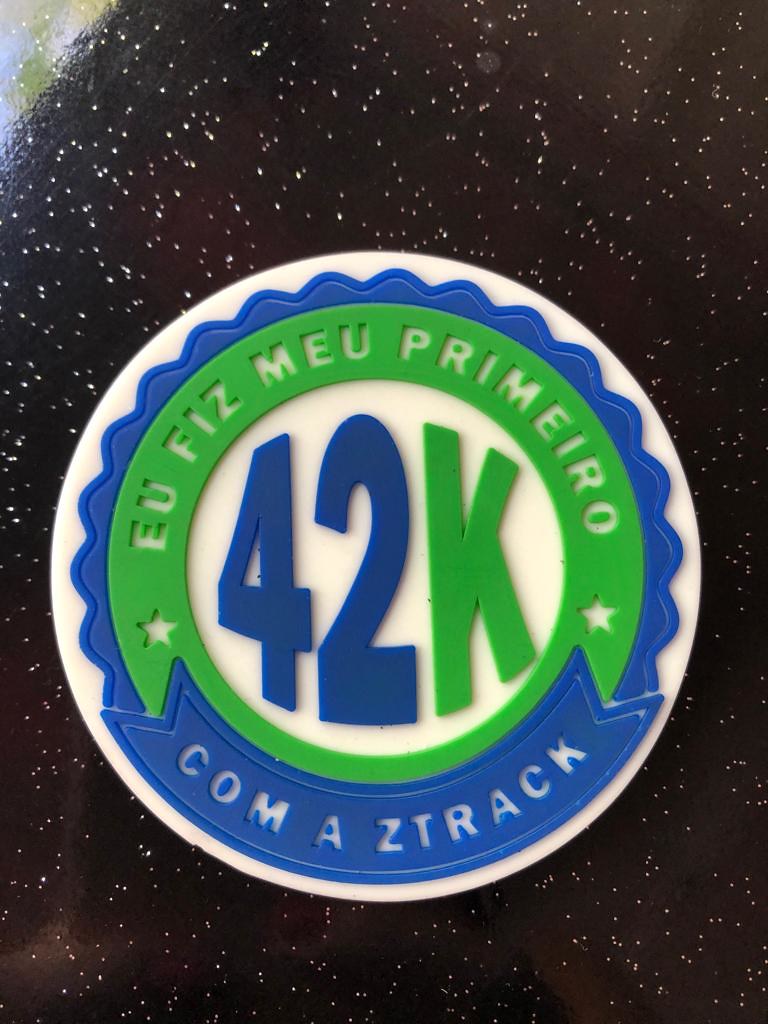This photograph features a uniquely designed medallion or possible refrigerator magnet that rests on a black tabletop accented with small, reflective silver flakes, creating an almost starry night effect. The medallion is a white circle, bordered by an intricate pattern of blue and green. A wavy blue ribbon encircles its lower half, forming a banner inscribed with "COMAZTRACK" in white letters. Within this border is a green ring, adorned at the top with the phrase "EUFIZMEUPRIMEIRO" and flanked by two blank stars. The core of the medallion showcases two large blue numbers, 4 and 2, positioned beside an equally prominent green letter K.